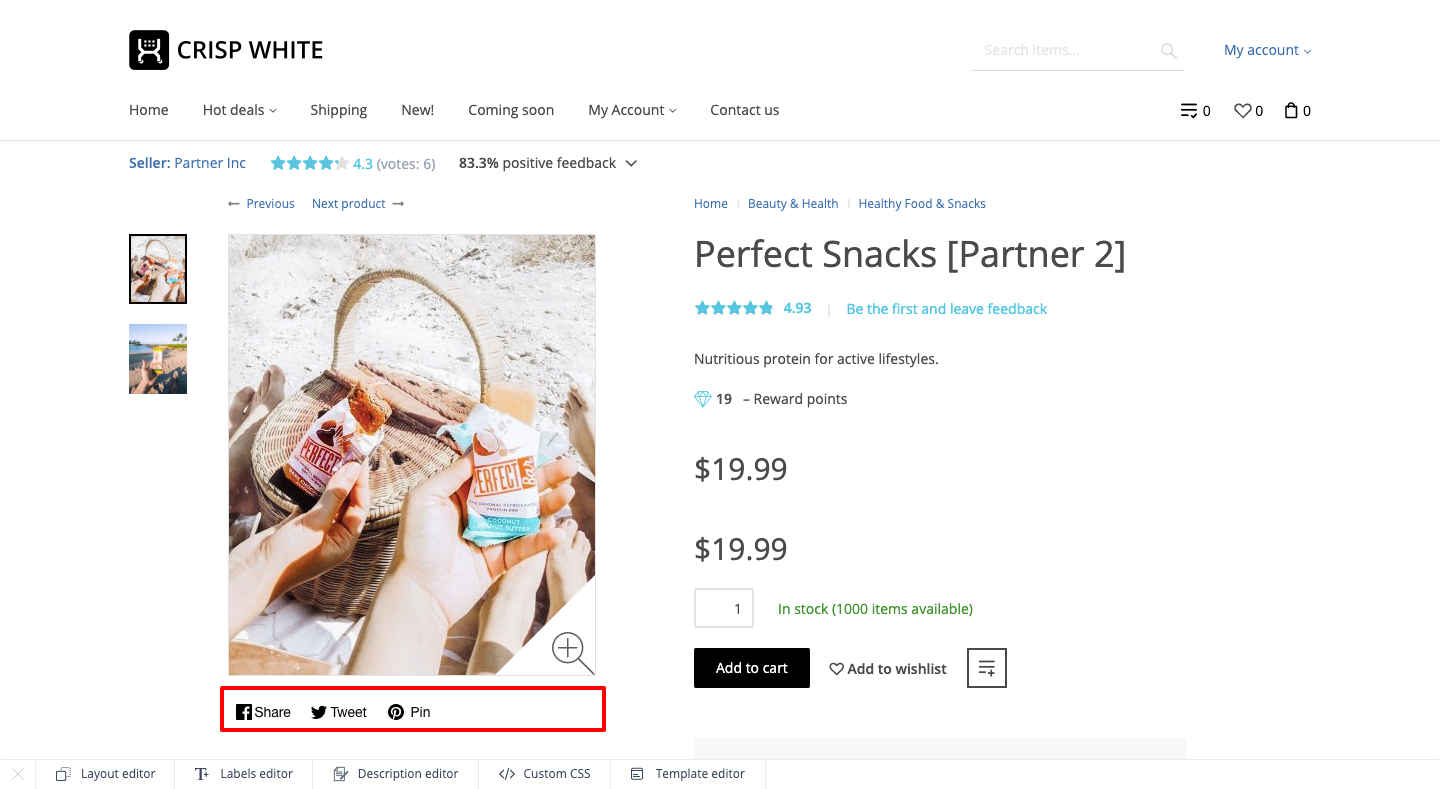The image depicts a detailed screen capture of a computer page. At the very top, the heading "Crisp White" is visible, accompanied by a distinctive icon located within a black box featuring a white illustrative design resembling an 'H' interspersed with dots. Just below this, there is a navigation bar with various clickable tabs arranged horizontally, directing users to different sections of the website. From left to right, the tabs read: Home, Hot Deals, Shipping, New!, Coming Soon, My Account, and Contact Us.

Progressing further down the page, there's an entry for a seller named "Partner INC." The seller boasts a rating of 4.3 stars out of 5, rendered in a teal color, with a note indicating that these ratings are derived from six votes. Additionally, the seller has an 83.3% positive feedback score.

Dominating the lower portion of the page is an image showcasing a person holding snacks nestled in a picnic basket. Below this image is a key product description that reads: "Perfect Snacks - Partner 2: Nutritious Protein for Active Lifestyles." The price for this product is listed as $19.99, and an adjacent black button allows users to add the item to their cart.